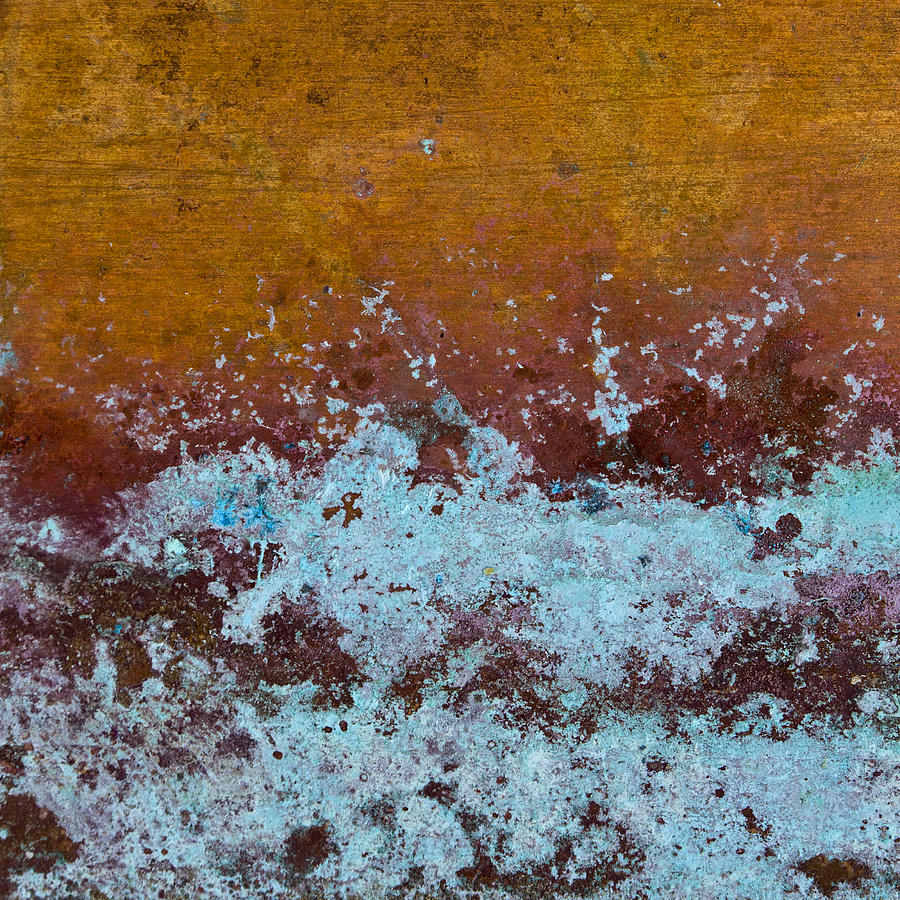The image features a striking and abstract composition that blends natural textures with vibrant colors, evoking both a sense of realism and artistic manipulation. The background appears to be a wooden table or board, possibly lacquered, displaying a gradient that transitions from light at the top to dark at the bottom. This wooden surface is overlaid with multiple layers of texture and color. 

Dominating the lower portion of the image is a rich, burgundy texture that has been splattered in an erratic pattern, mingling with a dark brown layer beneath it. Over this, a teal or light blue pigment spreads upward in a speckled spray-paint manner, creating an interplay between the colors. The teal hue is concentrated at the bottom, gradually dispersing and tapering off as it reaches higher.

The top part of the image features an orange-tan surface with horizontal scratch marks, resembling the rough texture of stone or rock. The overall impression is of a dynamic and layered scene, where the interplay of colors and textures—ranging from wooden grains and painted splatters to what may resemble mold or water damage—creates a captivating and complex visual experience.